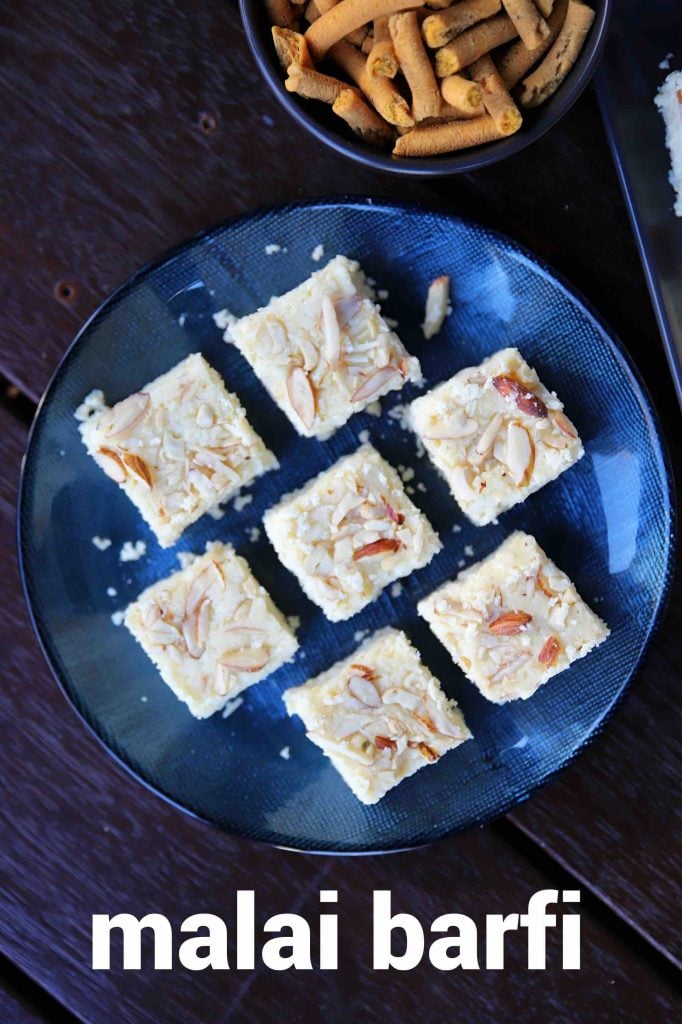The image showcases a dark, shiny wooden table as the background, with a centered blue plate displaying seven white confection squares known as Malai Barfi. The squares are arranged in a two-three-two pattern and are garnished with slivered almonds. Below the plate, white script reads "Malai Barfi." Above the plate, there's a matching blue bowl containing small brown, cylindrical treats resembling cinnamon sticks. Both the plate and the bowl feature a dotted design. The overall setting suggests a kitchen or dining area, with the confections and the bowl prominently placed in the center of the image.